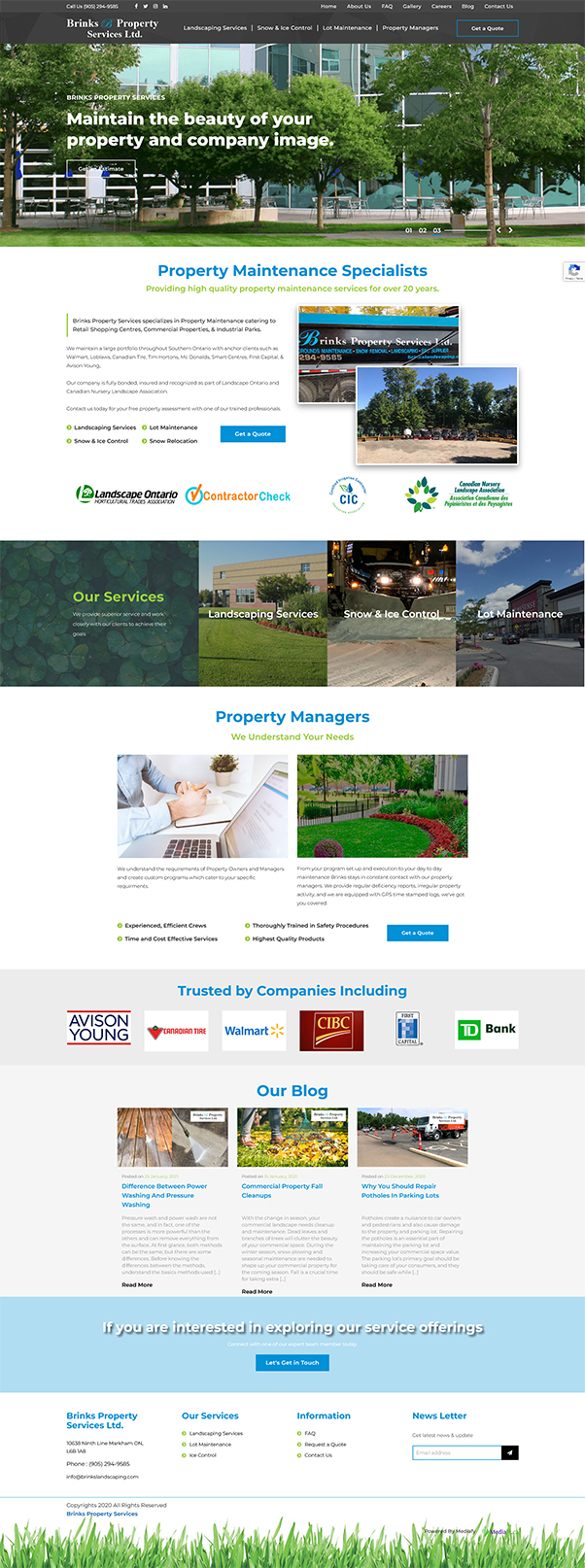A distorted, horizontally-stretched website showcases the extensive property maintenance services provided by Brinks Property Services Limited. The company prides itself on offering landscaping, snow and ice control, and lot maintenance services for over 20 years. Catering to retail shopping centers, commercial properties, individual parks, and industrial parks, Brinks specializes in maintaining the beauty of properties and enhancing company images. The site emphasizes their high-quality services, experienced and efficient crews, cost-effective and thorough procedures, and commitment to safety. It also highlights affiliations with organizations like Landscape Ontario and the Horticulture Association, assuring potential clients of their certified and reliable contractor status. Viewers are encouraged to get a quote for their tailored maintenance requirements.